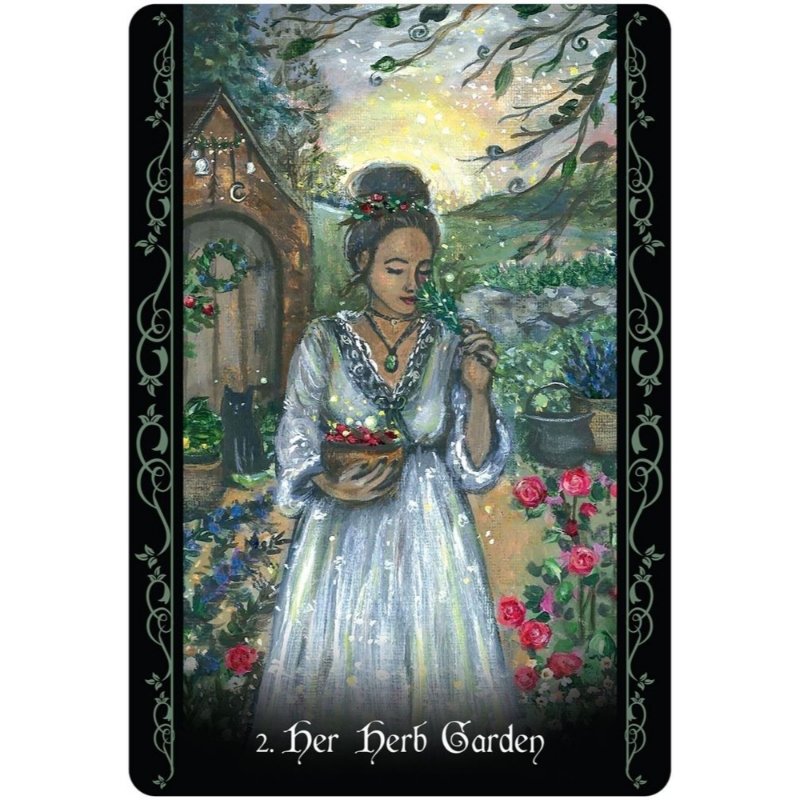The detailed illustration portrays a serene woman standing in her garden, bathed in the warm glow of either a rising or setting sun. She dons a flowing long white dress and has dark hair styled elegantly atop her head, adorned with red and green flowers. Around her neck hangs a black necklace with an oval green pendant. With her right hand, she delicately holds a bowl brimming with vibrant red flowers, while her left hand cradles a bunch of green herbs, which she gently smells with her eyes closed in peaceful appreciation. 

On the left side of the image is a black cat poised amidst an array of blue and red flowers. To the right of the woman, the garden continues to flourish primarily with red flowers, and in the background, a pot teeming with blue blossoms adds depth to the scene. This vertical rectangular piece, outlined by black strips with intricate silver designs along the edges, bears the inscription "To Her Herb Garden" at the bottom in white text. The scene hints at tranquility and self-contentment, encapsulating a moment of pure connection with nature.